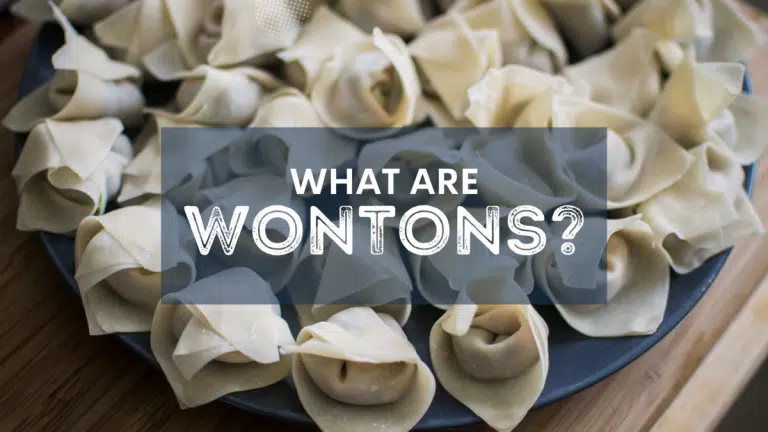The image is a high-resolution, color photograph in landscape orientation, capturing an exquisite presentation of wontons. The wontons, meticulously arranged in a circular pattern, fill a blue platter almost to overflowing. A translucent gray rectangle spans the middle of the image, providing a subtle overlay that reads, "What are Wontons?" in white text with a fine gray outline. The wontons appear handmade, suggesting a high-end culinary touch, perfect for soup. The platter rests on a light beige wooden surface, enhancing the overall warm and inviting aesthetic of the photograph. This image likely serves as an introduction to a magazine article exploring the origins, preparation methods, and various fillings of wontons.